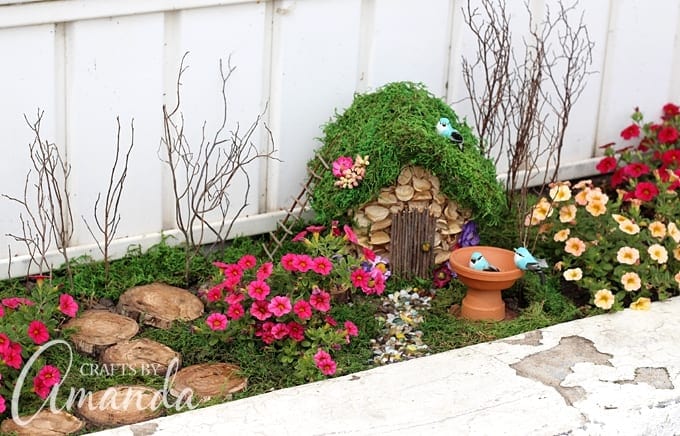This image is a detailed photograph of a meticulously kept small garden, akin to something from a home and garden magazine. On the lower left corner, there are a few small tree stumps or wooden plaques, cut into very small circles. The garden is adorned with a variety of flowers: pink on the left, yellow on the right, and red in the upper right corner. At the center, there’s a charming little wooden birdhouse with a door and a roof made of grasses. A miniature wooden ladder leads up to the roof, and atop the roof sits a small blue jay. In front of the birdhouse, there is a terracotta bowl acting as a bird feeder, with two blue and black birds; one is perched on the rim, while the other is inside the bowl. A small flower-lined pathway leads to the door of the birdhouse. The entire setup is framed by a white fence, with some stick-like structures resembling trees in the background, completing this quaint and inviting garden scene.